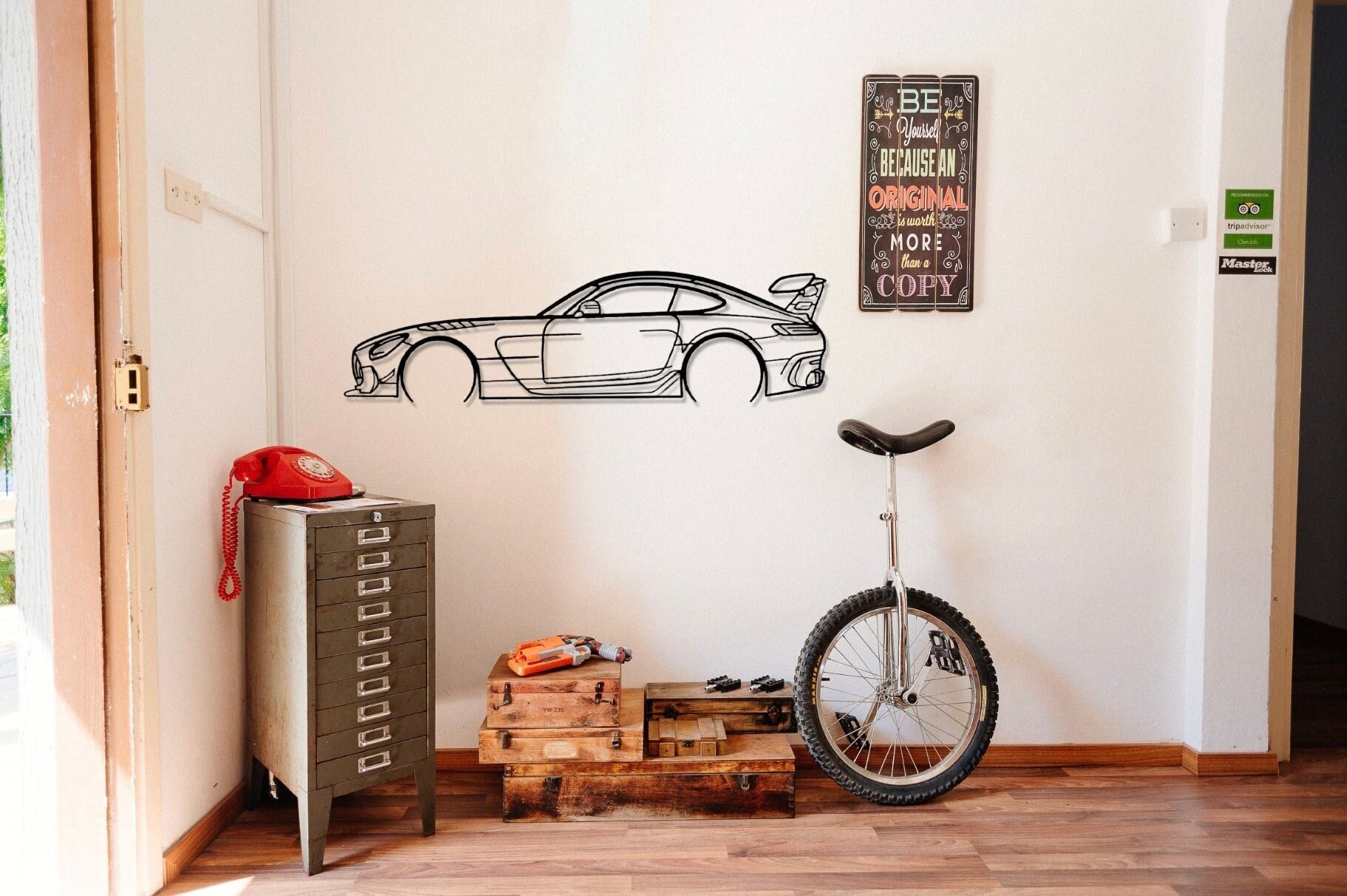This image depicts a sparsely decorated room within a house. Dominating the foreground, we see vinyl flooring featuring alternating light and dark brown panels. To the left, peeking in from the left edge of the image, the door frame is slightly ajar, revealing a touch of outdoor greenery. Inside the room, immediately to the left, stands a gray file cabinet about three feet tall with numerous drawers. Atop the cabinet rests a vintage red landline telephone reminiscent of those from the 70s and 80s.

The back wall of the room is painted white and showcases various decor. Prominently, there's a minimalistic wall art piece depicting the side view outline of a sports car without wheels, drawn in dark marker. Adjacent to it, a brown sign bears the motivational message: "Be Yourself. Because an original is worth more than a copy." Additionally, the room contains a unicycle leaning against the white wall, and a stack of wooden boxes or chests situated on the floor near the unicycle. The overall decor is minimalistic, focusing on a few key items and pieces of art.